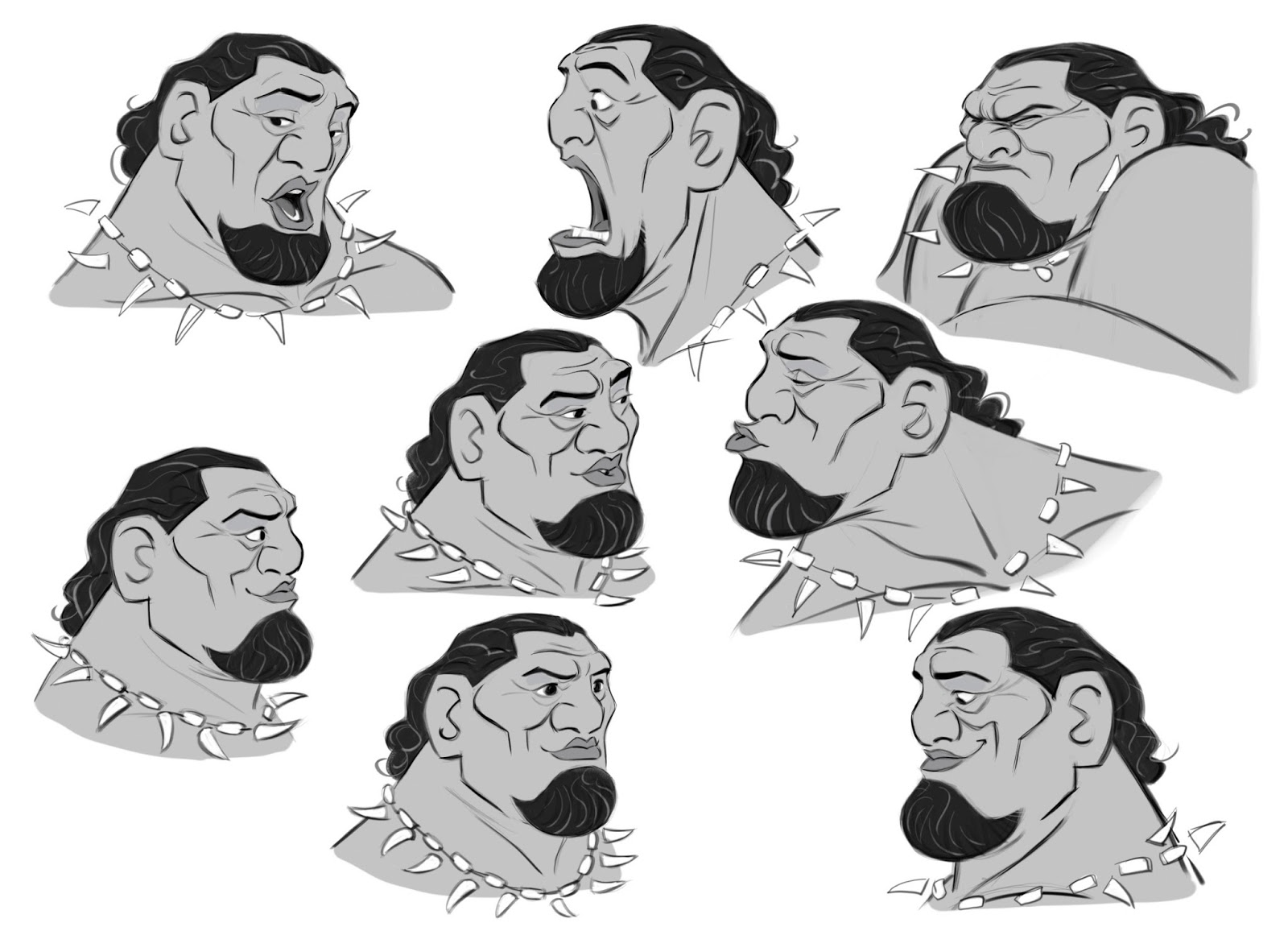The image features a series of eight black-and-white cartoon drawings of the same muscular man with long black hair, a short black beard, and a wide nose. His eyebrows are black, and he has full lips. The character’s face is large and masculine with sharp cheekbones and a distinct jawline. Around his neck, he wears a necklace adorned with what appears to be teeth or bones. The drawings showcase various emotional expressions: 

1. A surprised expression.
2. A shocked look.
3. Eyes tightly closed, seemingly not wanting to see something.
4. A smoldering expression.
5. A kissy face.
6. A profile view with a smile.
7. A diagonal angle smile showing more of his eyes.
8. A downward-facing smile showing just his profile.

The drawings capture a wide range of emotions, from excitement and sadness to mischievousness and pride. While the man's specific ethnicity isn't clear, he has features that could suggest a Pacific Islander or Samoan background. The illustrations focus only on his neck and above, accentuating his thick neck and robust build. Notably, the image is entirely monochrome, with no text, colors, or additional annotations.